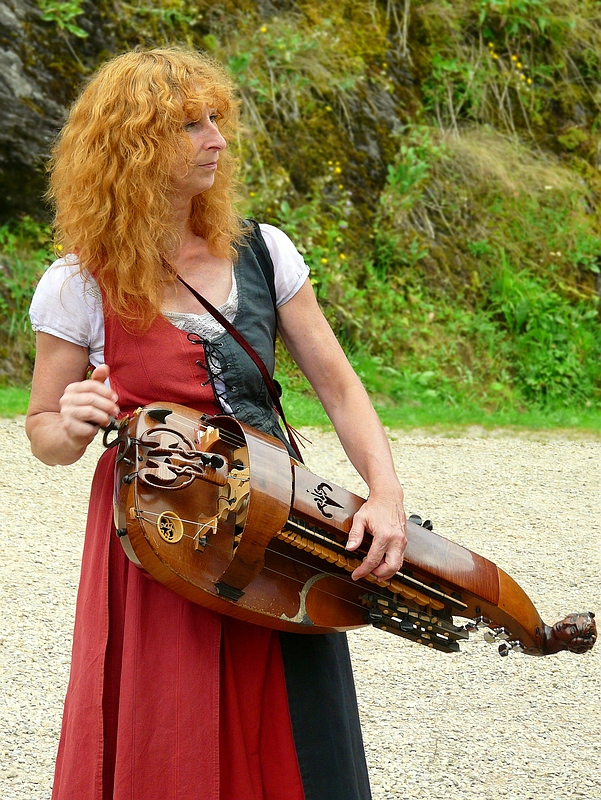The photograph captures a striking scene of a woman centered in the frame, visible from her knees upwards, holding and playing a large, ornate musical instrument known as a hurdy-gurdy. The rectangular photograph has a landscape orientation, with the length being twice the height. The woman, perhaps in her 30s to 50s, boasts voluminous, curly, ginger hair and is clothed in a unique and medieval-style outfit. Her dress is sleeveless, split with red on her left side and black on her right, laced at the chest with a black string through silver eyelets. Underneath the dress, she wears a short-sleeved, low-neckline white shirt. A thin brown leather strap crisscrosses over her shoulder, securing the glossy wooden hurdy-gurdy, which features a crank on one side and combines elements of both a piano and a guitar. She is performing in a natural outdoor setting, standing on light-colored gravel with lush greenery and hills in the background, under a cloudy sky.